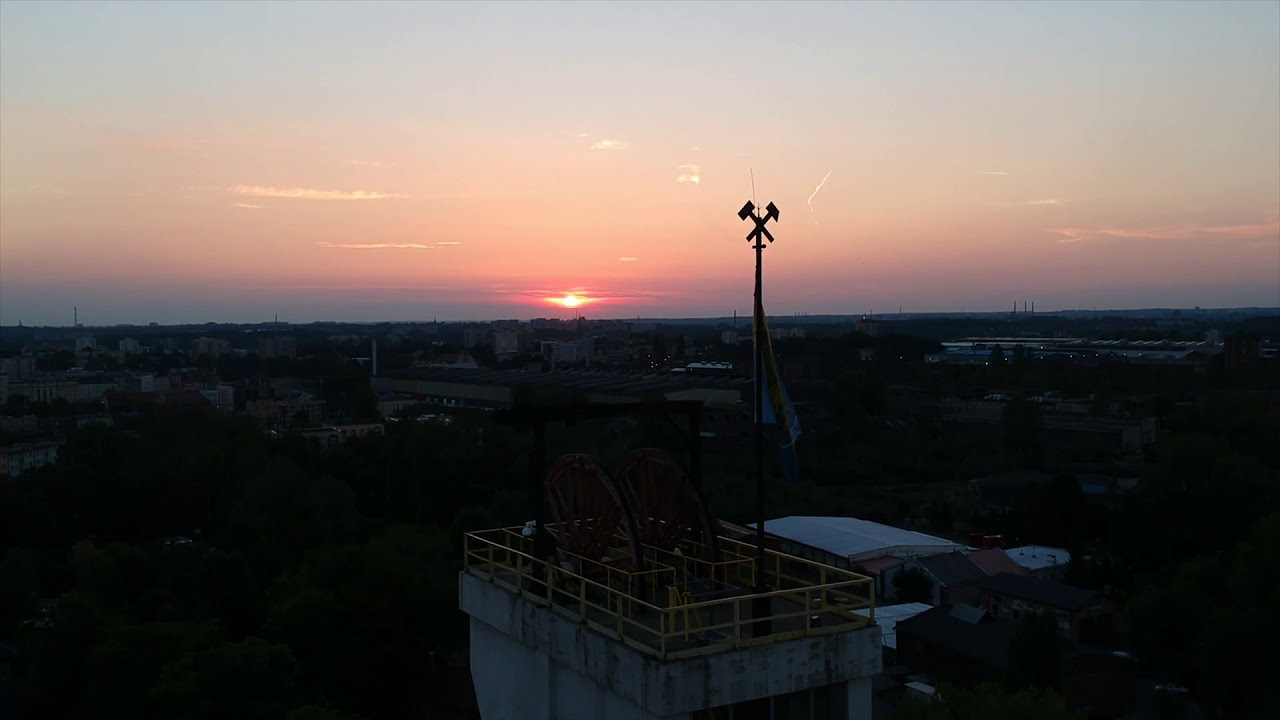This image captures an aerial view of a city at either sunset or sunrise, with the horizon line almost perfectly dividing the photo horizontally. The sun, slightly left of the center, is depicted with a round shape and two triangular jetting shapes giving it the appearance of having wings. The sky above the horizon is lit in a blend of reddish-pink and blue hues, with scattered white clouds. 

Dominating the middle of the photo is a prominent tower with a square base and surrounded by a yellow metal fence, resembling a radio or communication tower. The tower features a flagpole with a partially folded flag, showing hints of white and yellow, but the details are indistinguishable due to the dim lighting. At the top of the flagpole is an X-shaped metal structure with metal rectangles extending from each end.

The lower half of the image is very dark, making it difficult to discern details of the buildings. However, the tops of several structures are visible, including a large rooftop with two reddish wagon-wheel-like structures and various other buildings with flat roofs, antennas, and smokestacks scattered in the distance. Overall, the image beautifully captures the play of light and shadow at this transitional time of day, highlighting the city's skyline under the dawn or dusk sky.